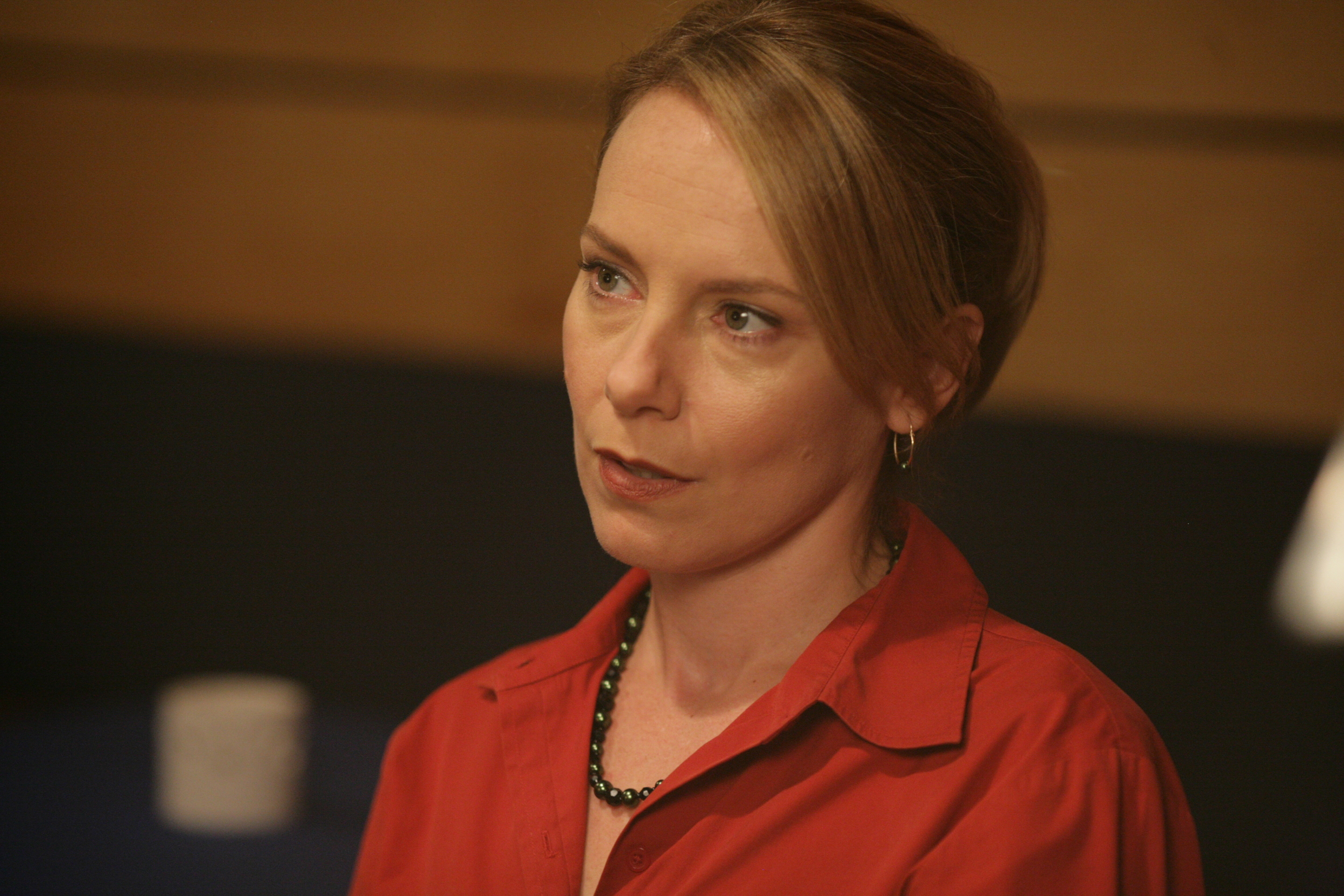The image is a very close-up photograph of a woman who appears to be in her late 40s or early 50s. She has light brown, almost blondish hair, which is either tied up or very short, not reaching her shoulders and styled with a slight comb-over in the front. She has a minimal makeup look, possibly just some eyeliner. Her attire includes a red V-neck or button-up collared blouse and a greenish beaded metal necklace. Additionally, she is wearing a thin metal hoop earring on her right ear. The background is blurred, predominantly black with a hint of a white object on the left side, which might be sitting on a seat. There might also be a wooden wall in the background. The expression on her face suggests she is either answering a question or about to say something important, conveying an inquisitive yet intense demeanor.